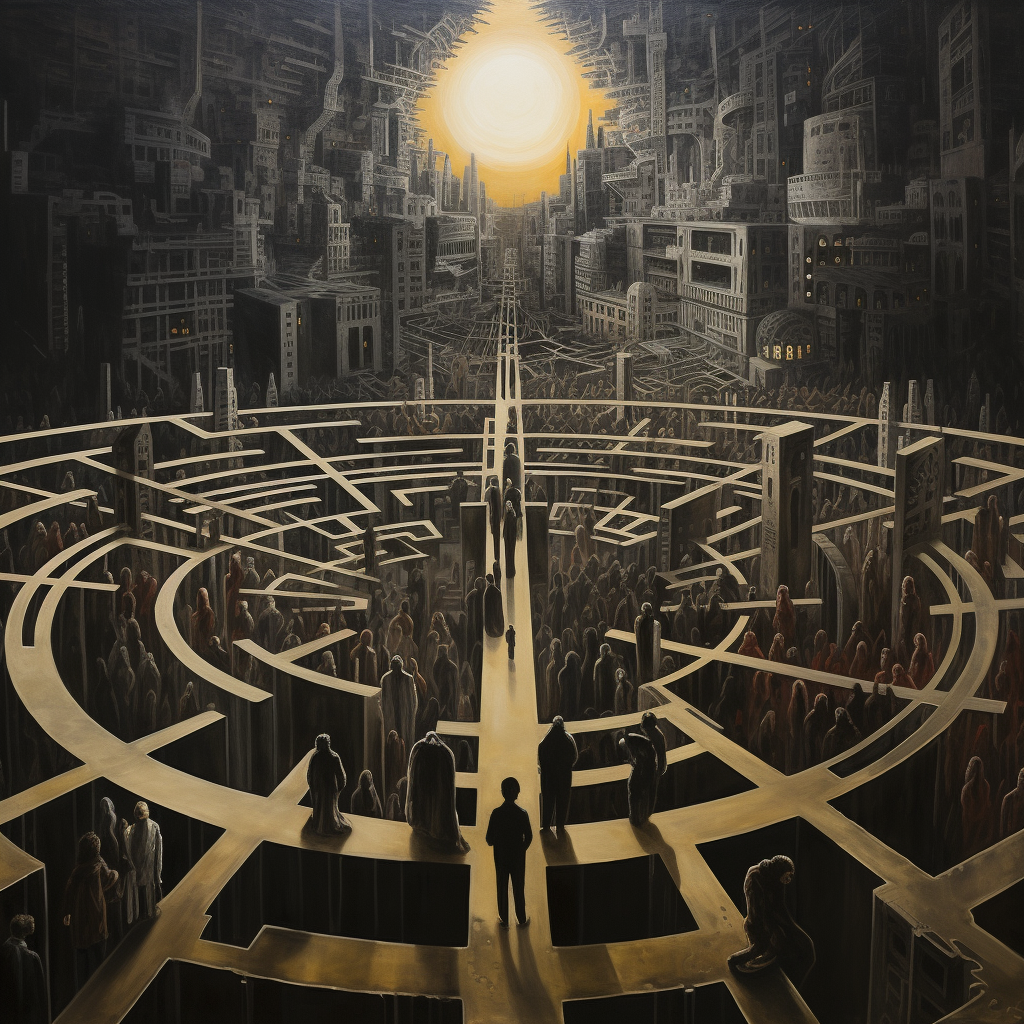The image depicts a striking, futuristic scene reminiscent of an M.C. Escher work. In the foreground, there's an elaborate maze-like structure constructed out of tall, metallic walls and concentric rings with intersecting lines. This labyrinth features both elevated pathways and lower ground sections. Indistinct figures populate the maze, with some walking along the elevated walls that form the labyrinth, while others navigate through the pathways below. A prominent pathway extends from the bottom center of the image, rising to meet the middle of the frame, suggesting a continuous journey. The entire maze is bathed in a goldish hue that contrasts with the grayscale cityscape in the background. This cityscape is dense with modern skyscrapers, contributing to the overall sci-fi aesthetic. Dominating the background, a bright orange sun peeks through an opening at the top center of the maze, casting a surreal glow over the scene. The combination of the intricate maze and the futuristic cityscape creates a mesmerizing and detailed visual experience.